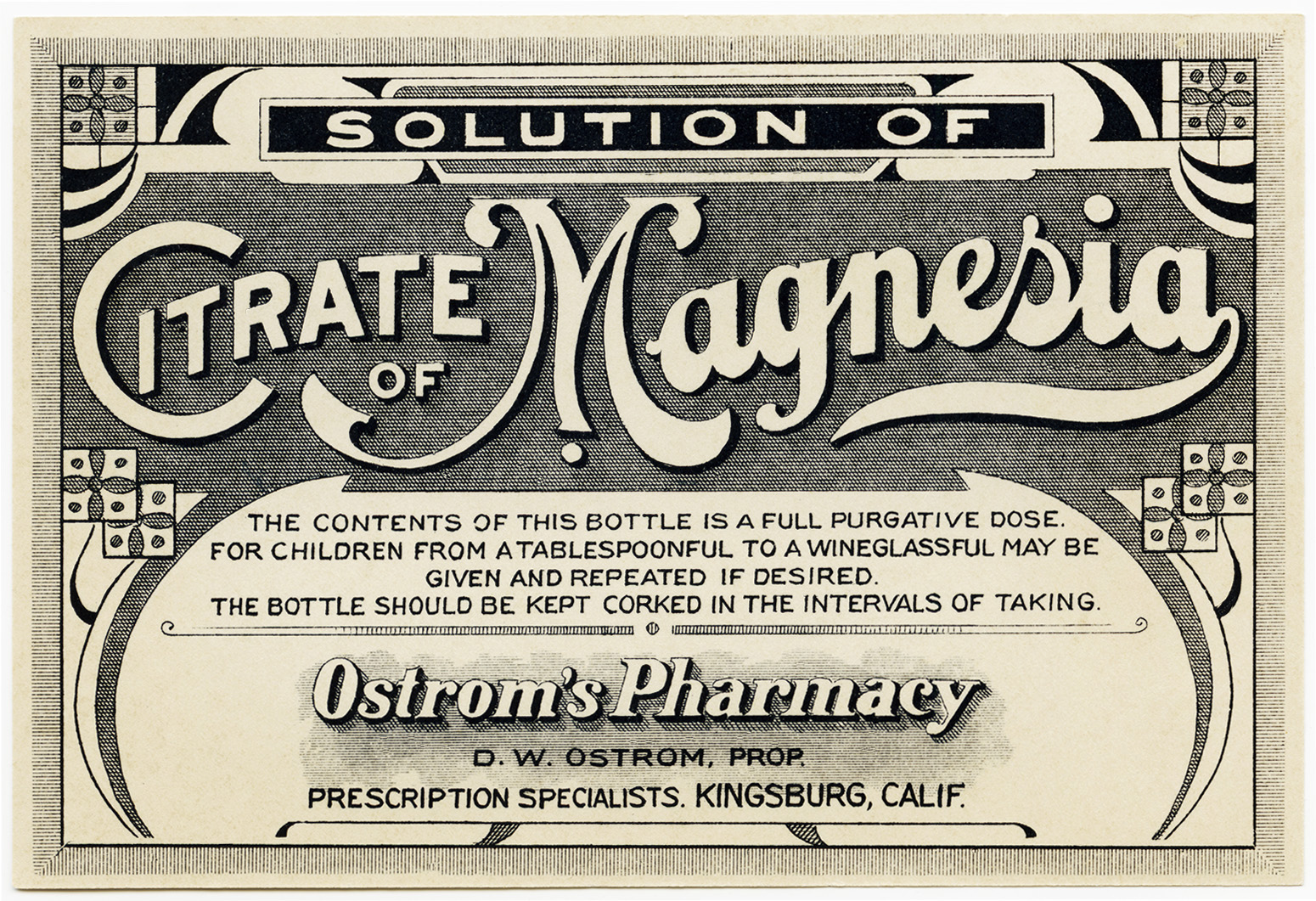The image is a grayscale scan of an old printed label related to a pharmacy. The label features various intricate details. At the very top, there's a black bar with white letters reading "Solution of." Below this, in the center, on a gray background, the text "Citrate of Magnesia" is prominently displayed in a very large, curvy, and stylized font. The text “Citrate of Magnesia” is notably detailed, especially the letter "M," which appears particularly ornate. Further down, on a white background with black letters, the label states, "The contents of this bottle is a full purgative dose. For children, from a tablespoonful to a wine glassful may be given and repeated as desired. The bottle should be kept corked in the intervals of taking." Toward the bottom, in large white letters, it reads "Ostrom's Pharmacy," and in smaller text, the details "DW Ostrom PROP, Prescription Specialist, Kingsburg, California" are provided. Additionally, there's a decorative floral design with dots at each top corner, adding to the vintage appearance of the label.